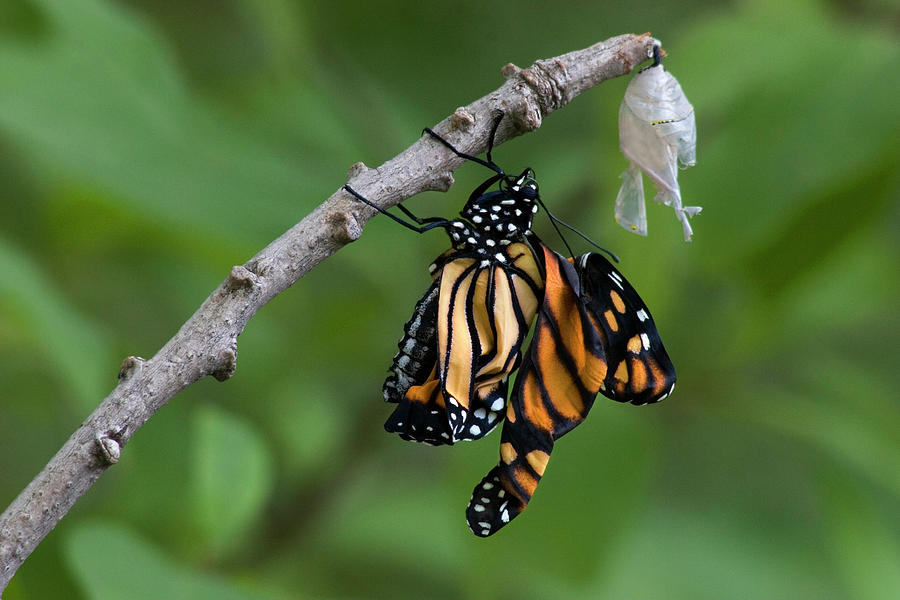This vivid color photograph captures a close-up of a monarch butterfly freshly emerged from its chrysalis. The butterfly clings to a slender, arched brown branch stretching from the bottom left to the upper right of the image. Its wings, still not fully expanded, display a striking pattern of orange with black lines and white spots, while its black body is also adorned with white spots. The butterfly's front legs grip the side of the branch, and its back legs wrap around it, giving the impression that the butterfly is hanging upside down as it adjusts to its new form. At the very tip of the branch, to the upper right of the frame, hangs the torn, light-gray chrysalis from which the butterfly has just emerged, resembling delicate paper. The background is a blend of blurred, indistinct shades of green, enhancing the photograph's focus on the detailed beauty of the monarch and its former cocoon.